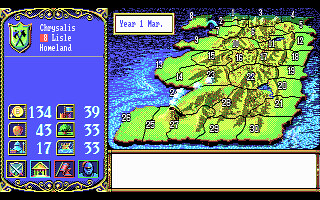This is a detailed still image from a video game, depicting an in-game map. The map background is blue, highlighting a prominently green map that resembles a county map, with regions clearly defined by thin black lines and numbered for easy identification. The map intricately displays mountainous terrain and diverse landscapes, adding depth to the visual depiction of the area. On the left side of the image, there is a vertical rectangle in periwinkle blue, bordered with a gold trim. At the top of this rectangle, the words "Chrysalis," "Lazelle," and "Homeland" are inscribed. The upper left corner of the rectangle features a small green coat of arms depicting two crossed axes. The bottom section of the rectangle includes various numbers and legend icons, which likely serve as a guide to understanding different elements and regions on the map.